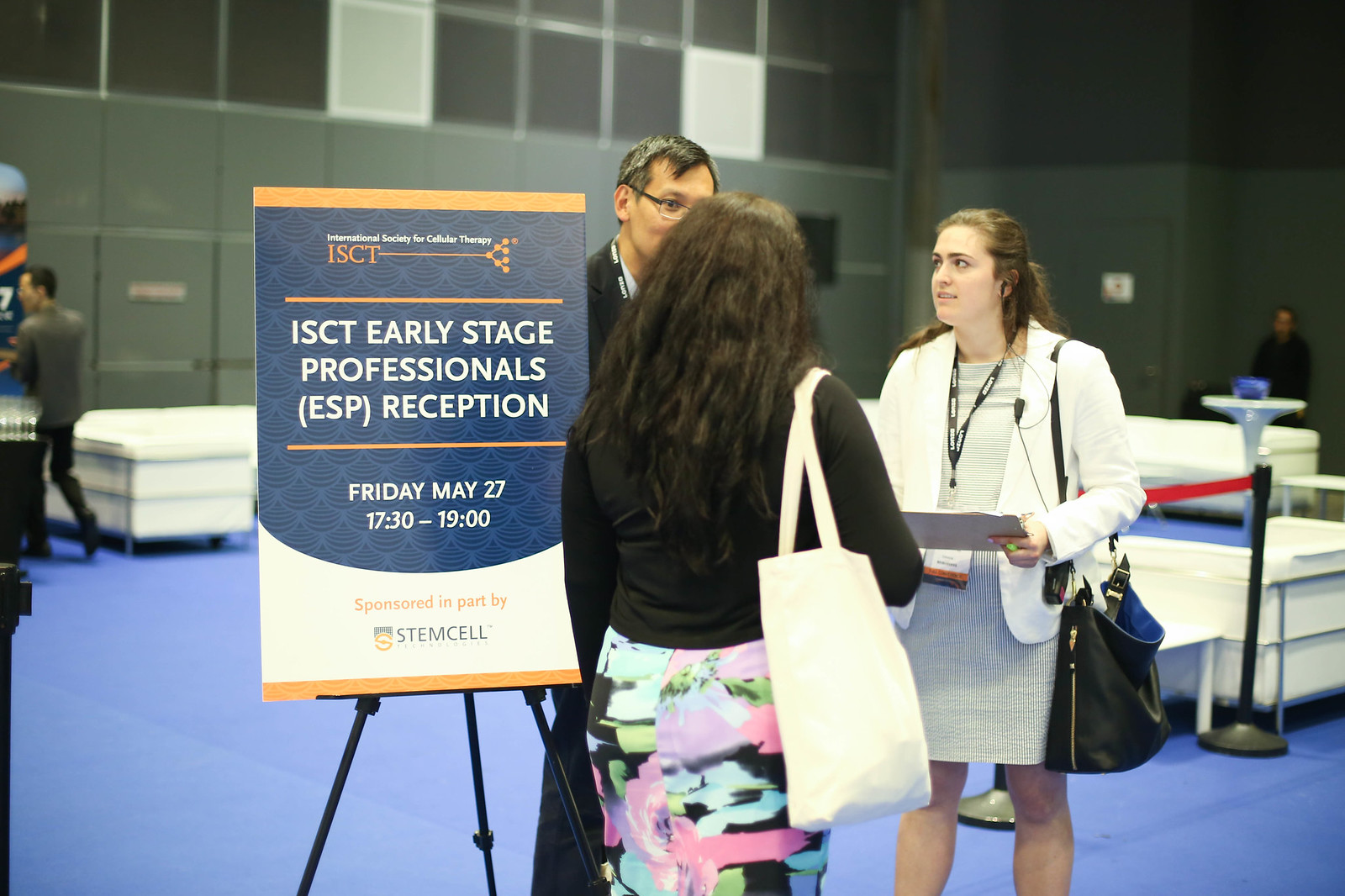This color photograph, taken inside a large auditorium or convention center, captures a moment at the International Society for Cellular Therapy (ISCT) Early Stage Professionals Reception, held on Friday, May 27th from 1730 to 1900 hours, and sponsored in part by StemCell. Three individuals are the focal point of the image. In the foreground, a woman with long wavy dark hair stands with her back to the camera. She is wearing a long-sleeved black shirt and a colorful skirt with shades of pink, blue, and black, and has a white tote bag on her right shoulder. She faces a man and a woman who appear to be engaged in conversation with her. The woman facing the camera sports straight brown hair and is dressed in a black and white dress paired with a white jacket. She carries a black tote bag on her left shoulder and holds papers in her hand. To her left, a middle-aged man with short, graying dark hair and glasses is partially visible. He is dressed in a dark suit consisting of a black top and black slacks. Behind them, the spacious room has blue carpeted floors, gray and black walls, and high ceilings. A blue sign near the group displays event details, while the background reveals white tables, containers, and scattered attendees.